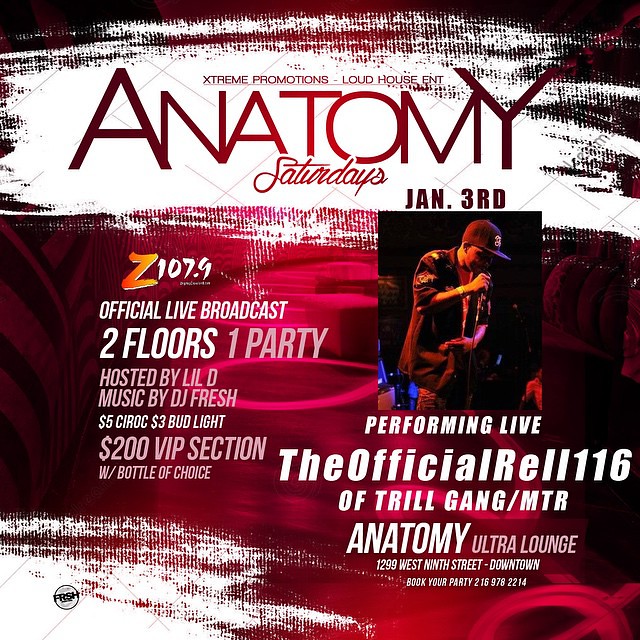This digital event flyer, featuring a bold red and black abstract background, promotes "Anatomy Saturdays" set for January 3rd at the Anatomy Ultra Lounge. At the top, in striking crimson red letters, it announces the live performance of the official REL 116 of Trill Gang/MTR. The flyer prominently showcases a black-and-white photograph of the performer looking down at a crowd, wearing a flat-brimmed black cap and a black shirt. It highlights key details like the Z107.9 Original Live Broadcast and the "Two Floors, One Party" theme, hosted by Lil D with music by DJ Fresh. Additional event perks include $5 Siroc, $3 Bud Light, and a $200 VIP section with bottles of choice. The flyer also provides the lounge’s address at 1299 West 9th Street, Downtown, and booking information at 216-978-2214.